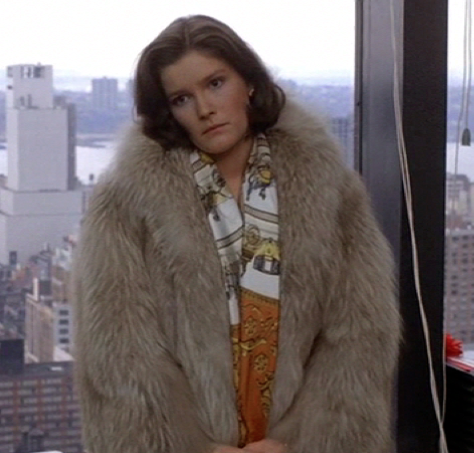This is a detailed, older-looking photograph, possibly from the 1990s, featuring Kate Mulgrew, the renowned actress known for her role as the captain on Star Trek: Voyager. She is standing on the upper level of a tall building, likely in New York City, given the visible skyline and buildings below and in the distance. The background includes a hazy sky, suggesting an elevated height that offers a panoramic view of the cityscape, including distant rooftops and what might be a hint of a lake.

Kate Mulgrew is attired in a striking, large fur coat that blends off-whites, browns, and grays. Beneath the fur, she is wearing a colorful shawl or scarf that has a predominantly white pattern with yellow drawings and a brown horizontal stripe, along with an orange section at the bottom, perhaps adorned with paisley designs.

Her shoulder-length brown hair, parted towards her left eye, frames her serious, unsmiling face as she slightly tilts her head to the right, almost looking down but with eyes directed ahead. She stands next to a window with a metal pillar on the left side, suggesting she is positioned at the corner of the building. Threads appear to be coming around her from the left side, adding to the scene's complexity and hinting at a sophisticated, almost cinematic ambiance.